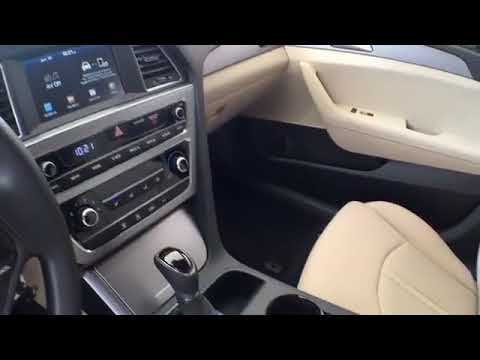The image is a small, horizontally aligned rectangle with thick black borders at the top and bottom, showcasing the interior of a vehicle from the front seat perspective. Prominently featured is the console which includes a digital screen at the top, a clock displaying the time as 10:21, various dials for the heat and air conditioning settings, the hazard light button, and the radio controls. Below these elements is the gear shifter, gray with a black top, and part of a cup holder. The picture captures just the edge of the black steering wheel on the far left. On the right side, the interior door panel is visible in the upper right-hand corner, along with part of the light tan or white leather passenger seat and the white interior of the door frame. The glove box and part of the window side area are visible, with the black floor area at the bottom.